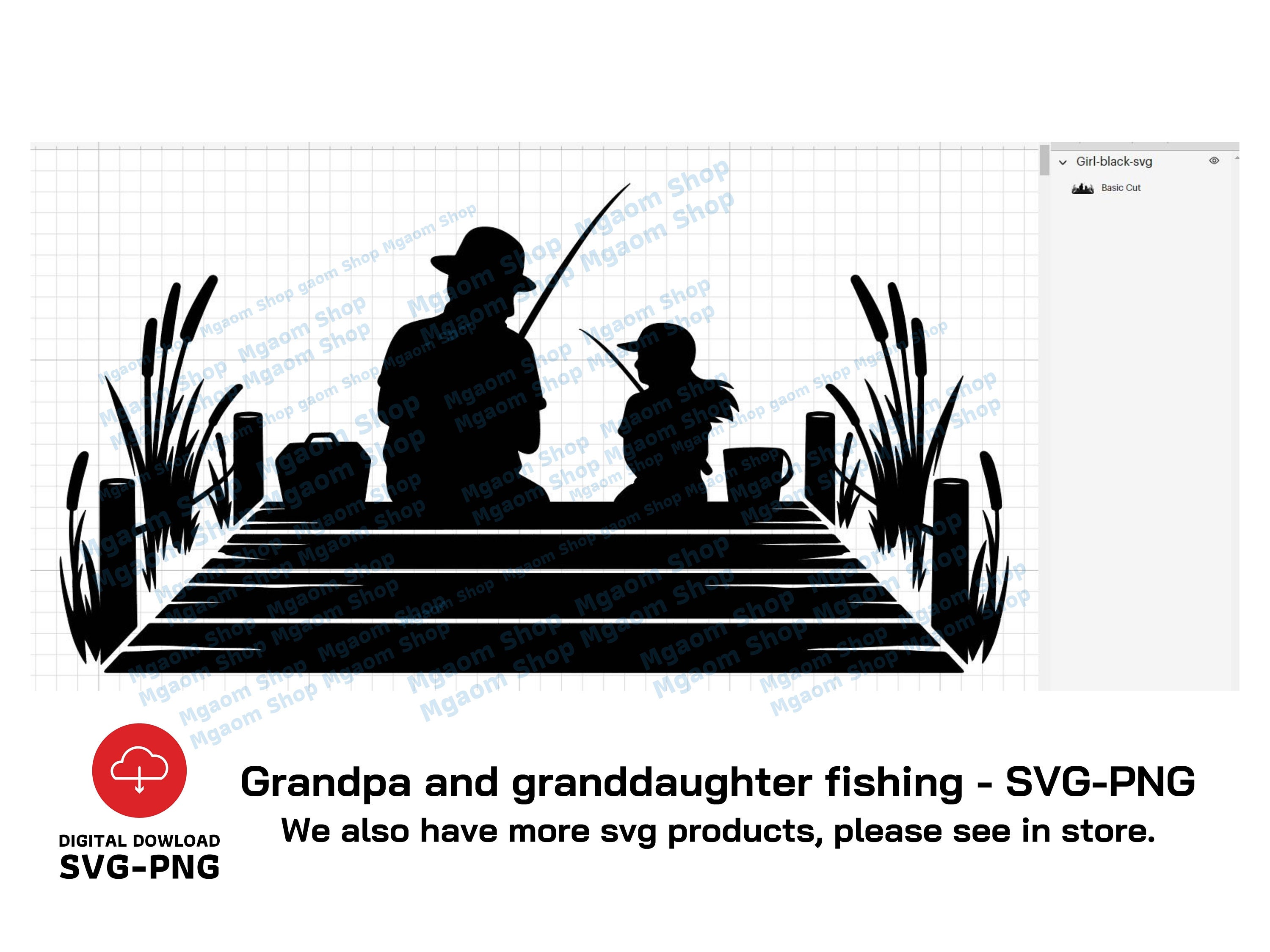The image is a digital download available in SVG-PNG format, depicting a touching scene of a grandpa and granddaughter sitting on the edge of a pier, fishing together. The entire scene is rendered in silhouette, emphasizing their figures and the outlines of their fishing gear against a serene backdrop. The adult, wearing a hat, holds a fishing pole and has a tackle box nearby, while the little girl, with her hair flowing, clutches a smaller fishing pole and has a pail beside her. The black silhouettes contrast beautifully with the white gridded background, enhancing the peaceful and nostalgic mood of the image. Additional details include plants beside the pier, two rows of promotional text at the bottom, a watermark in blue text overlaying the grid, and a red cloud icon in the bottom left corner. A gray sidebar on the right side of the screenshot lists the file name and presents a down arrow for download, labeled "basic cut." This enchanting scene occupies about 75% of the upper middle portion of the image.